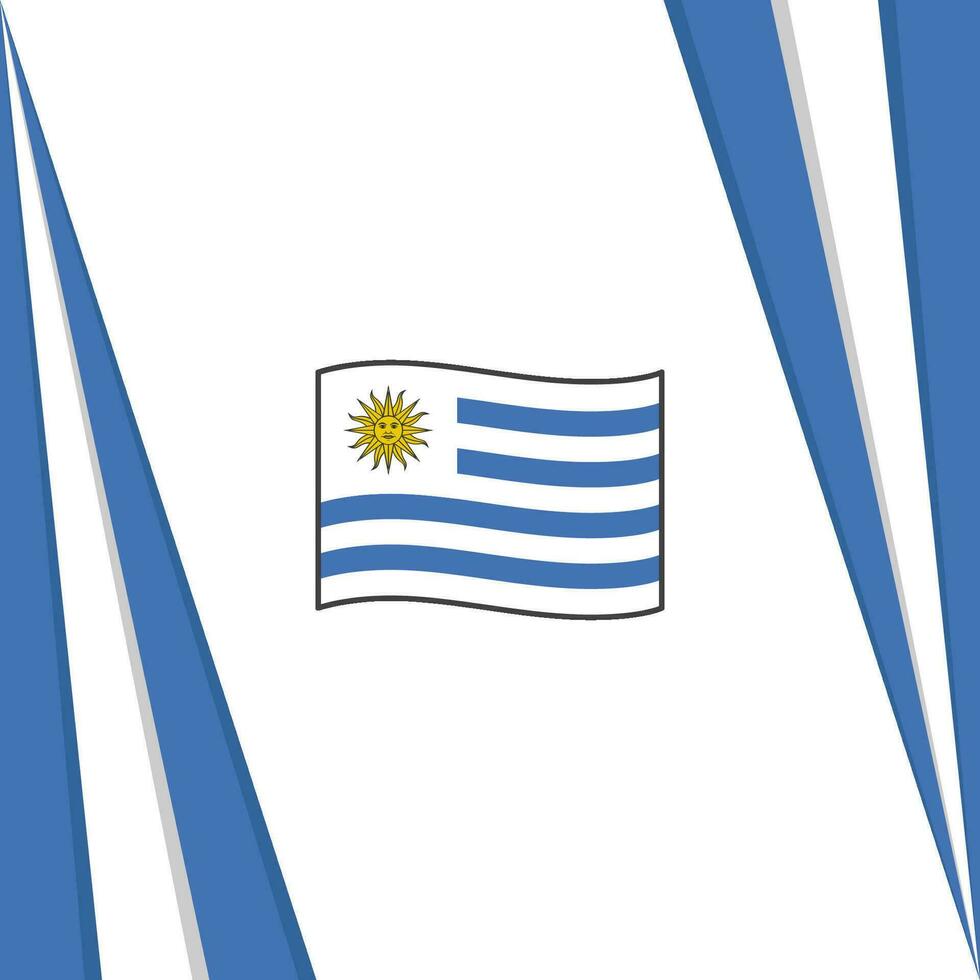This detailed image appears to be a computer-drawn or cartoon depiction, primarily featuring the colors white, blue, and yellow. It is structured within a square canvas. On this canvas, there are two sets of prominent blue triangles positioned at opposite corners. The first blue triangle extends from the bottom left corner to the top left corner, while the second blue triangle extends from the top right corner to the bottom right corner. These triangles are separated by a central white area, forming a striking geometric pattern.

At the heart of the image, occupying the central position, is a flag. The flag itself is white with four horizontal blue stripes, two of which are shorter and located at the top and the other two longer ones at the bottom. To the left of the two shorter stripes, filling the top left portion of the flag, is an outlined sun icon with a face, characterized by two eyes, a nose, and rays emanating from the center—all outlined in black.

The overall composition creates a visually balanced design with blue, white, and yellow as the dominant colors.